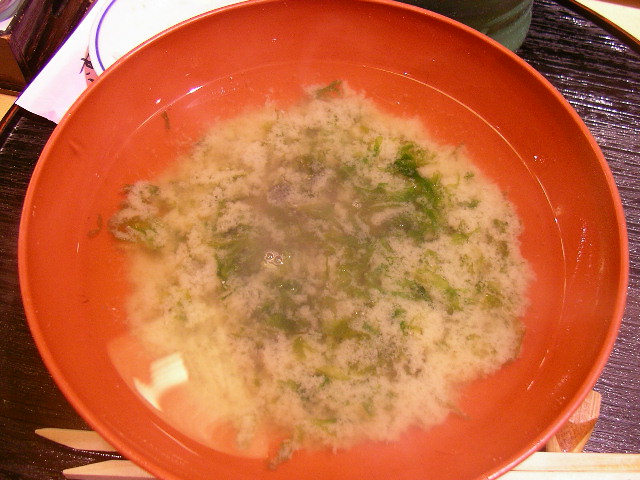The photograph, taken from directly overhead, features an eye-catching orange bowl set on a shiny, dark brown, striated table. The bowl, possibly made of plastic, contains a liquid that transitions from clear at the top to a cloudy white near the base. Suspended within the liquid are green accents, possibly vegetables, and brown spots that might be pieces of meat. Reflecting the flash from the camera, the bowl dominates the image. In the foreground, partially obscured by the bowl, are the tips of what appear to be wooden chopsticks. In the background, to the upper left, lies the edge of a white plate with blue trim and a piece of paper, possibly a menu, featuring a graphic of a shrimp.